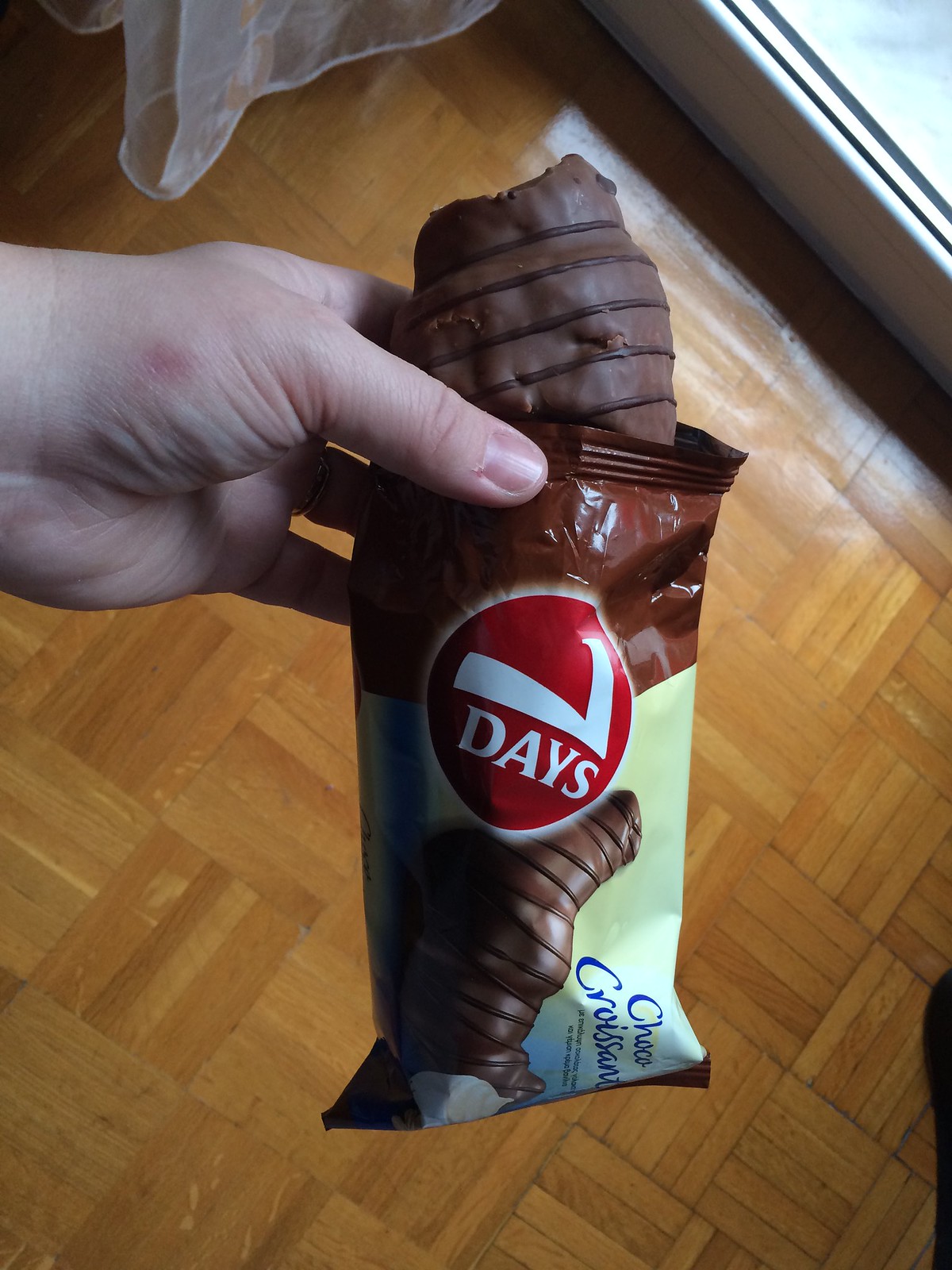This photograph captures a close-up of an opened package featuring a chocolate croissant, held by a pale-skinned left hand with neatly trimmed nails and a lesion on the palm. The packaging prominently displays the brand name "7 Days" in white lettering on a red circular background. The label at the bottom of the pack includes an image of the chocolate croissant alongside the text "Choco Croissant." The wrapper transitions from a brown color at the top to a light white color at the bottom. Emerging from the opened package, the chocolate croissant itself appears delicious, showcasing decorative darker chocolate drizzles across its top. A bite has been taken out of the croissant, revealing a partly eaten interior. The background features a medium brown parquet wooden floor with a crisscross pattern that gives a synthetic tile appearance. Additional details include an electric baseboard heater, a sheer curtain, and light shining through the bottom of a window in the upper right corner of the image.